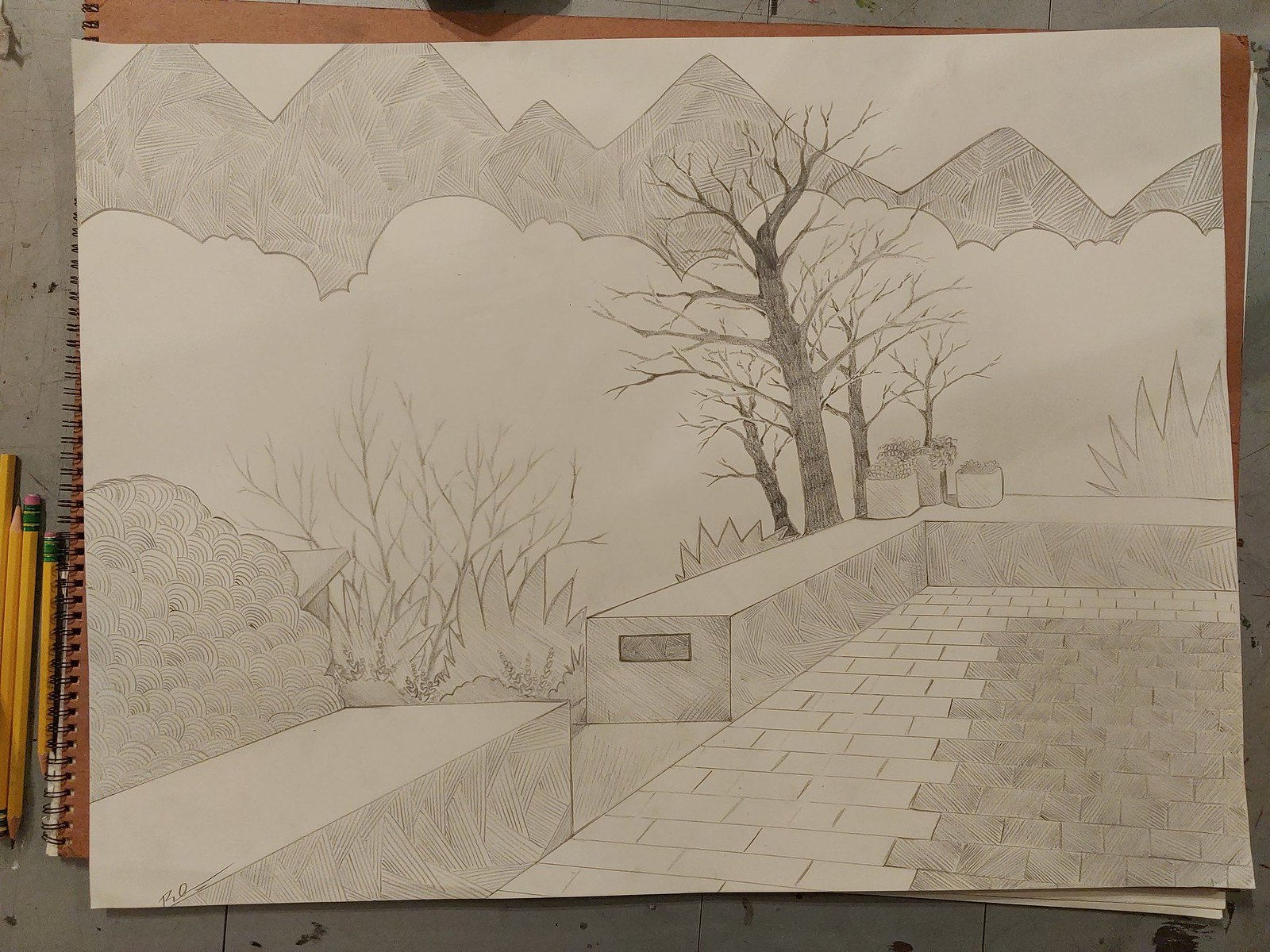This intricate black-and-white illustration, meticulously rendered in pencil on a large piece of white paper, depicts a serene outdoor setting. On the left side of the scene, lush, detailed bushes create a sense of depth and natural beauty. Adjacent to them, a quaint bench invites viewers to imagine sitting and basking in the tranquility of the environment. 

Atop small pedestal-like structures, an arrangement of three pots, each containing a plant, adds an element of curated nature and human touch to the scene. Behind this arrangement stands a large, leafless tree, its branches intricately sketched to reveal their stark beauty. Flanking this central tree are three smaller trees, also devoid of leaves, their bare branches creating an intricate network against the sky.

Beneath the large tree, a variety of bushes, drawn in triangular patterns, add a textured layer to the composition. In the background to the left, a mixture of dead trees introduces a somber note to the otherwise peaceful landscape. Beyond these, a delicate outline of distant clouds and a majestic mountain range provides a breathtaking backdrop, completing the scene with a sense of vastness and quiet solitude.